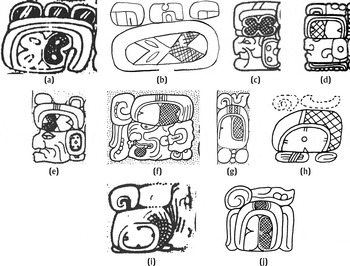The image comprises ten black-and-white illustrations labeled with lowercase letters from "a" to "j." These sketches appear to be parts of what might form a totem pole when stacked together. The drawings showcase a mix of intricate designs and facial depictions. Four of the illustrations depict elaborate faces with strong features—such as defined noses, aged wrinkles, prominent chins, and traditional headdresses—while the remaining six contain abstract and curvilinear designs. Notably, illustration 'a' features a complex arrangement including three bulbous shapes on top and a swirling pattern below, resembling a butterfly with contrasting black and white halves. Each subsequent illustration combines unique elements like block letters, crosshatchings, and ovals. The faces oriented to the left include individuals with varying degrees of age and expression. Together, these sketches create a cohesive yet varied collection that suggests an artistic representation of cultural icons often found in totemic imagery.